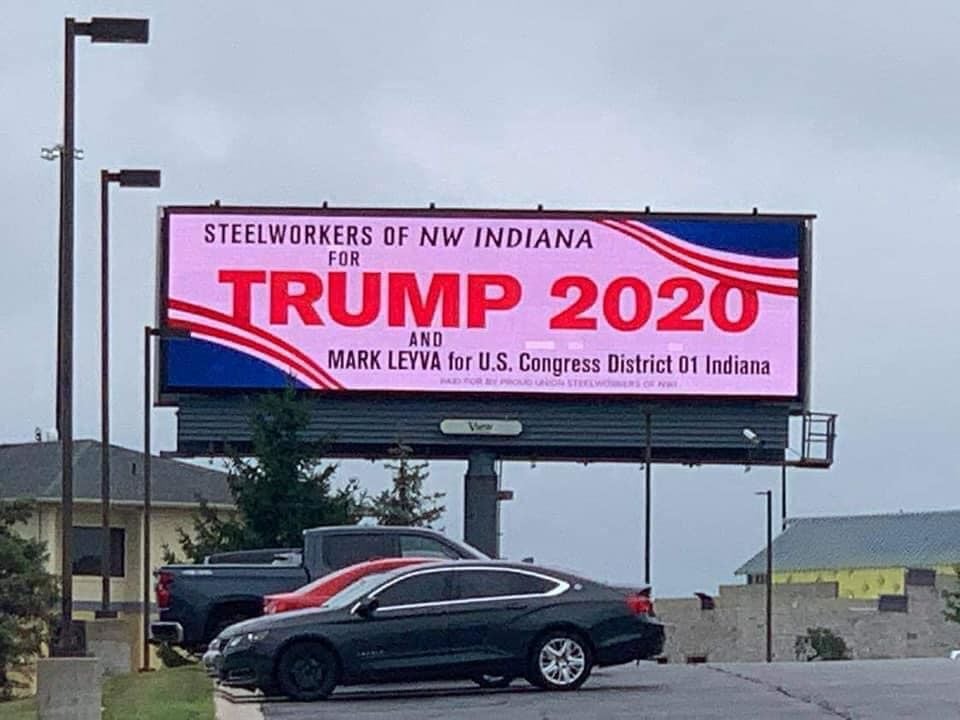The image depicts a large, illuminated billboard at the back of an asphalt parking lot. The billboard prominently features a campaign message that reads "Steelworkers of Northwest Indiana for Trump 2020" in large bold red text, with additional text below endorsing Mark Leyva for U.S. Congress, District 01, Indiana. The design includes subtle pink background tones with red and blue stripes in the upper right and lower left corners. In the foreground, several late-model cars are parked, flanked by green grass and trees indicating a likely summer or early fall setting. Street lights illuminate the parking area, casting subtle glows on surrounding structures. To the left, there is a cream yellow building with large picture windows, while a brick building with a gray roof is visible further in the background. The overall scene is set against a gray, overcast sky, with some construction visible in the distance.